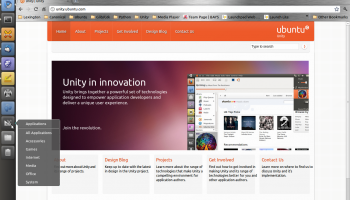A detailed caption for the image described could be:

"A screenshot taken from a PC showcasing the Unity Innovation interface on an Ubuntu operating system. The visible section is titled 'Unity Innovation,' although the accompanying icons are quite small and difficult to discern. The text above clearly reads 'Ubuntu.' The image contains several elements, but the finer details and inscriptions are not legible."